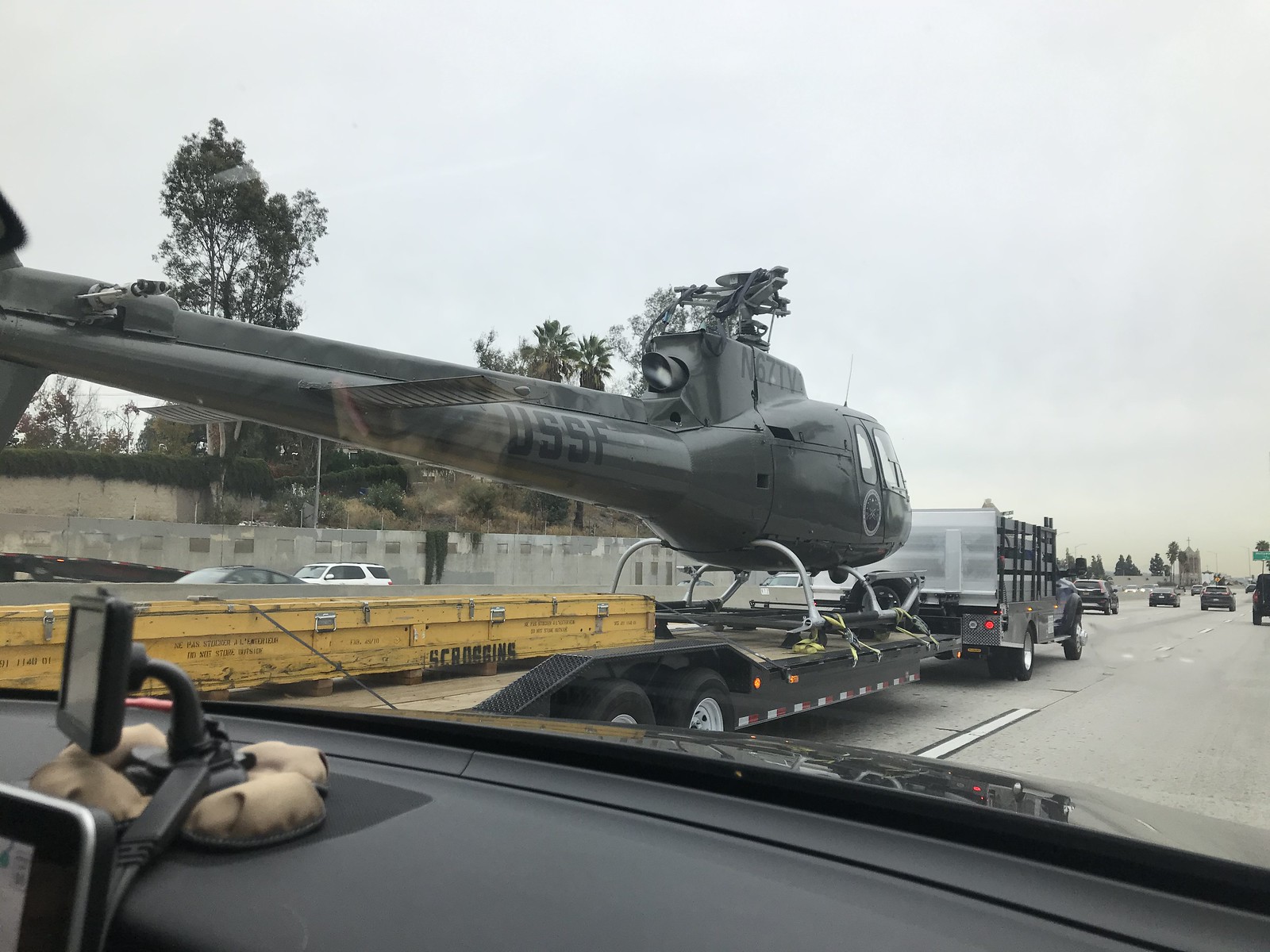In this daytime photograph taken from the perspective of a passenger sitting inside a car, we see the road ahead through the windshield. Notably, in the adjacent lane, a military helicopter is being transported on a long, multi-wheeled trailer pulled by a truck. The helicopter, painted in military green with "USSF" marked on its tail, features a pod-like body and an extended tail. Its rotors have been removed for transportation. The trailer carrying the helicopter is brown and yellow. The car from which the photo is taken has its dashboard and camera visible. Surrounding traffic includes several cars traveling in both the same and opposite directions, emphasizing the dynamic setting.